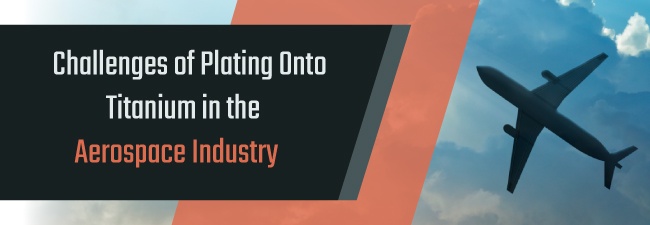The image is a horizontal advertisement for the aerospace industry. Featured prominently on the right side is the underside of a passenger airplane set against a blue sky filled with various clouds. The sky has a bluish tint with some areas showing white clouds, indicating a clear daytime setting. Towards the center, there is a slanted orange parallelogram, creating a bold visual element. On the left side of the image, more clouds are visible towards the bottom with a bit of blue sky peeking at the top. Overlaying these elements is a black trapezoid on which the text is displayed. The white text reads, "Challenges of Plating Onto Titanium in the" followed by "Aerospace Industry" in striking orange letters, matching the color of the central orange shape.